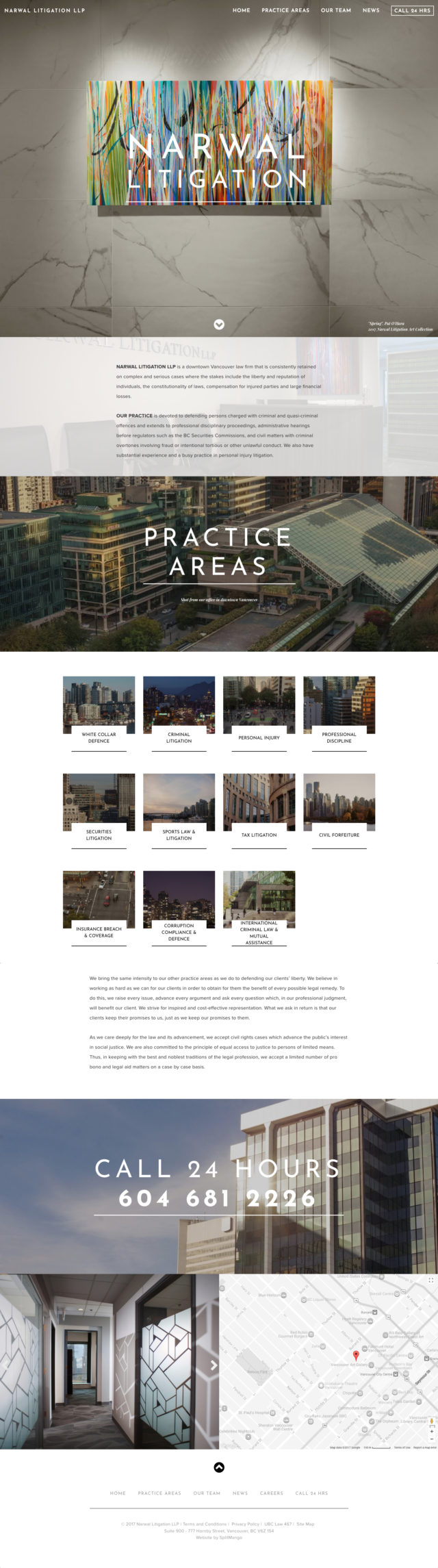The image consists of a vertically extended display featuring multiple sections, each meticulously detailed. At the very top, there is a gray marble background composed of neatly fitted tiles. Nestled in the middle of this marble backdrop is an elegant piece of artwork that reads "Narwhal Litigation."

Beneath this section, a column of text is divided into two paragraphs. Directly below the text, there is another photo. This part of the image seems to pertain to "Practice Areas," which is followed by an arrangement of smaller images.

These smaller images are organized into three rows. The first and second rows each contain four photos set side by side, while the third row holds only three photos. This is followed by an additional two-paragraph text section.

At the bottom of the image, there is another notable photo. The top portion of this photo prominently displays the text "24 hours 604-681-2226." This photo is split into two distinct images in the lower half: the left side depicts a long hallway, and the right side features a hand-drawn map.

This detailed layout effectively conveys complex information through a series of visually organized elements, making it easy to navigate and understand.